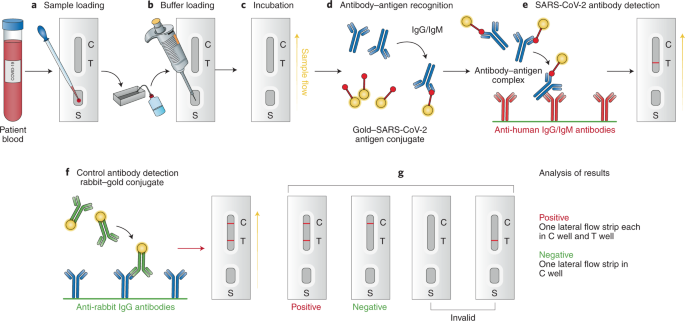This image is a detailed scientific diagram illustrating the process of blood testing for SARS-CoV-2 antibodies, depicted in multiple stages from A through G. Set against a white background, it begins in the upper left with a vial of patient blood, recognizable by its red contents and blue cap. To the right, step-by-step procedures are organized in gray boxes.

- **A: Sample Loading** - The blood sample is loaded onto a small applicator or tester.
- **B: Buffer Loading** - A syringe is used to add a buffer to the applicator.
- **C: Incubation** - The sample incubates to enable reactions.
- **D: Antibody-Antigen Recognition** - Y-shaped antibody molecules and antigen conjugates (depicted as little yellow and red circles) interact.
- **E: SARS-CoV-2 Antibody Detection** - The antibody detection is shown through a test strip marked with 'C' (control) and 'T' (test) wells. A red line indicates a result.
- **F: Antibody Detection, Rapid Gold Conjugation** - More detailed detection steps with red lines appearing by the 'C' and 'T' indicators.
- **G: Analysis of Results** - The outcomes are evaluated as positive (lines in both C and T wells), negative (line only in C well), or invalid (no line or a line only on T well).

Throughout the diagram, various antibody and antigen interactions are depicted with colored Y-shaped objects and lines, highlighting the biochemical processes involved. The bottom row reiterates the critical final analysis where the presence or absence of lines determines the test result.